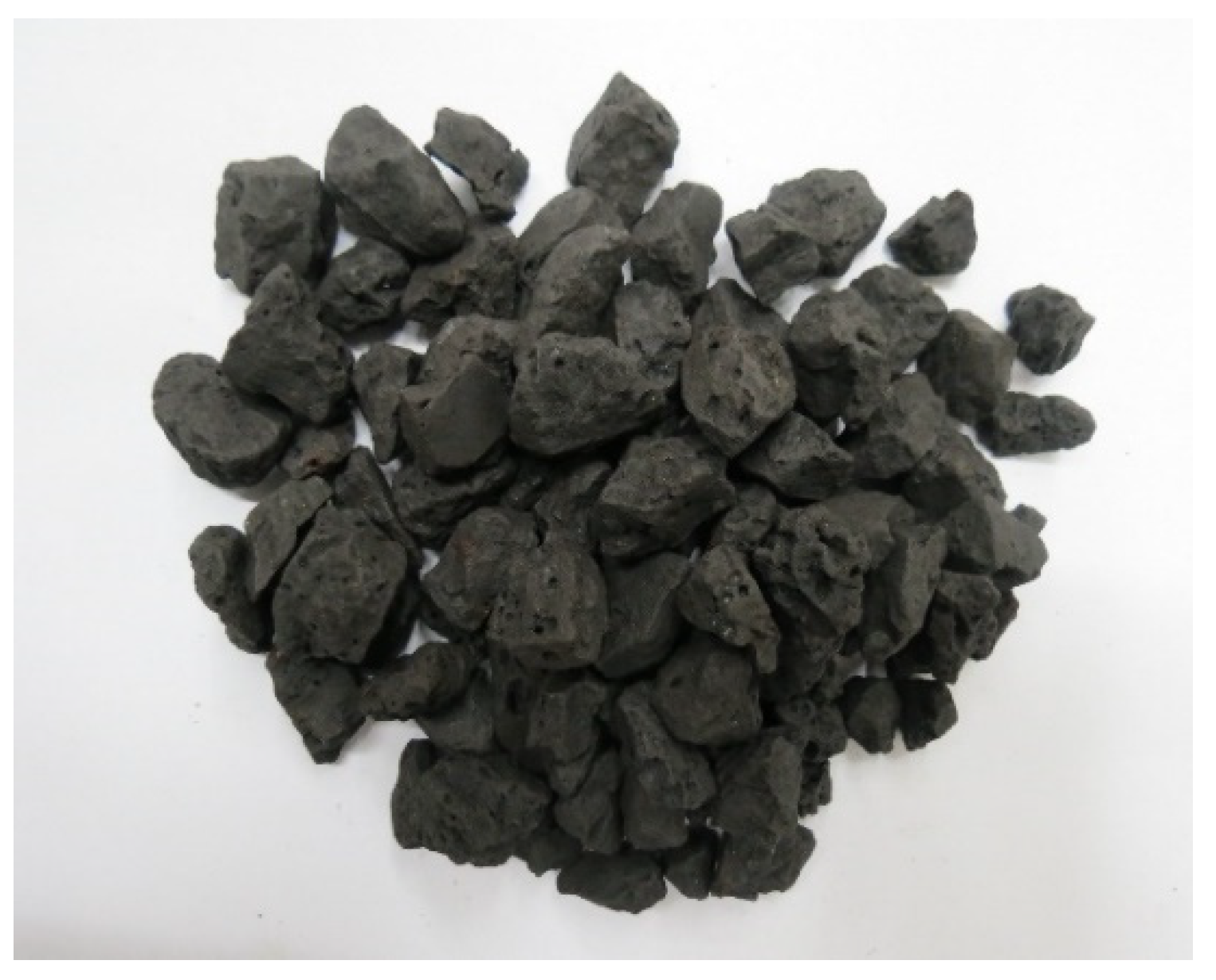The image is a black and white photograph, rectangular in shape, with the longer side being horizontal. The background is predominantly white with subtle shadows. Central to the photograph is a pile of about 50 to 60 craggly, dark gray to black rocks, likely basalt or another volcanic rock. The rocks are roughly shaped, uneven in size, with the largest rock being approximately five times the size of the smallest. They range from about an inch to two inches in diameter and feature sporadic small holes, hinting at their porous nature. The rocks are somewhat loosely arranged in a heart-like pile, with a few scattered around the main cluster, and their shadows are visible on the white backdrop.